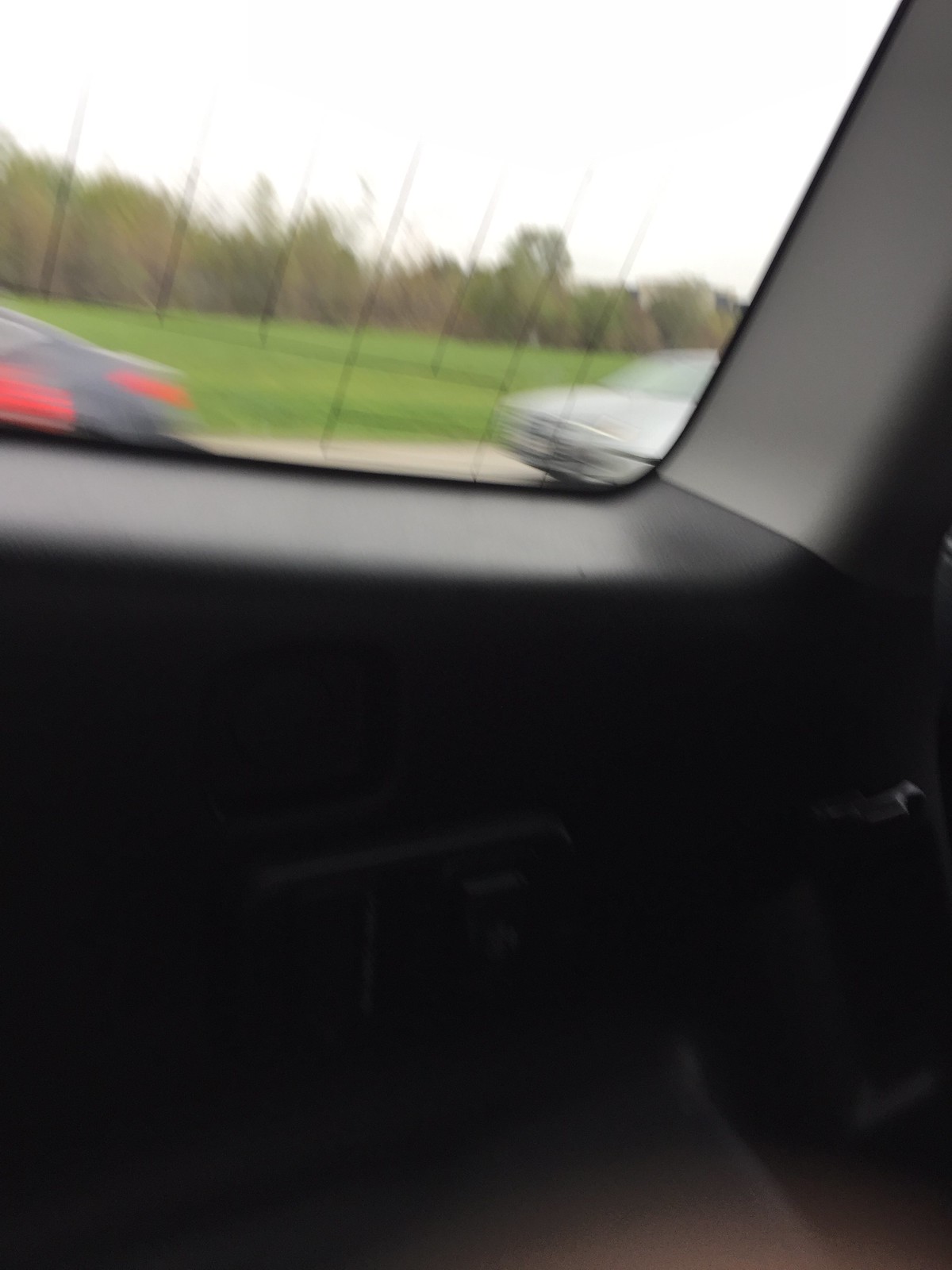The image, taken from inside a vehicle, captures a slightly blurred interior scene. Key details include one of the vehicle’s side windows, featuring an up-and-down button for window control, and part of the handle and floorboard, all rendered in black. The window shows faint lines, likely antenna lines embedded in the glass. Beyond the window, there's a view of green grass and two passing cars: a silver car with a blurred front, possibly headlights, and a black car with red taillights and a distinctive red stripe. The backdrop consists of a grassy field leading to a cluster of trees, under a sky that appears almost white.